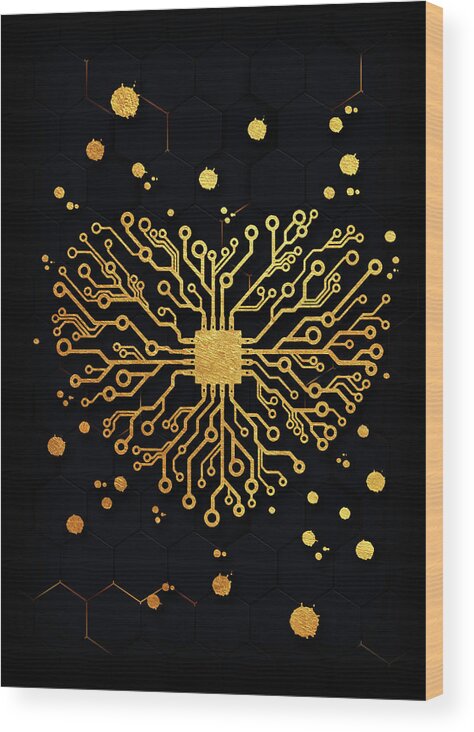The artwork depicted in this image is a rectangular piece with a light brown edge, oriented slightly to the left, revealing its dimensions and depth. The main feature of the piece is a digital heart at its center, set against a black background adorned with a subtle honeycomb pattern. The heart is constructed from intersecting straight lines and adorned with golden dots at their endpoints, creating a striking visual network reminiscent of a computer chip. This digital heart features a central square, from which various lines and wires extend in multiple directions, culminating in gold circles that define the heart's boundary. Subtle zigzag patterns can be observed both at the top and bottom of the artwork, adding to its intricate design. The overall composition seamlessly blends technological aesthetics with artistic elements, highlighted by the interplay of black and gold tones.